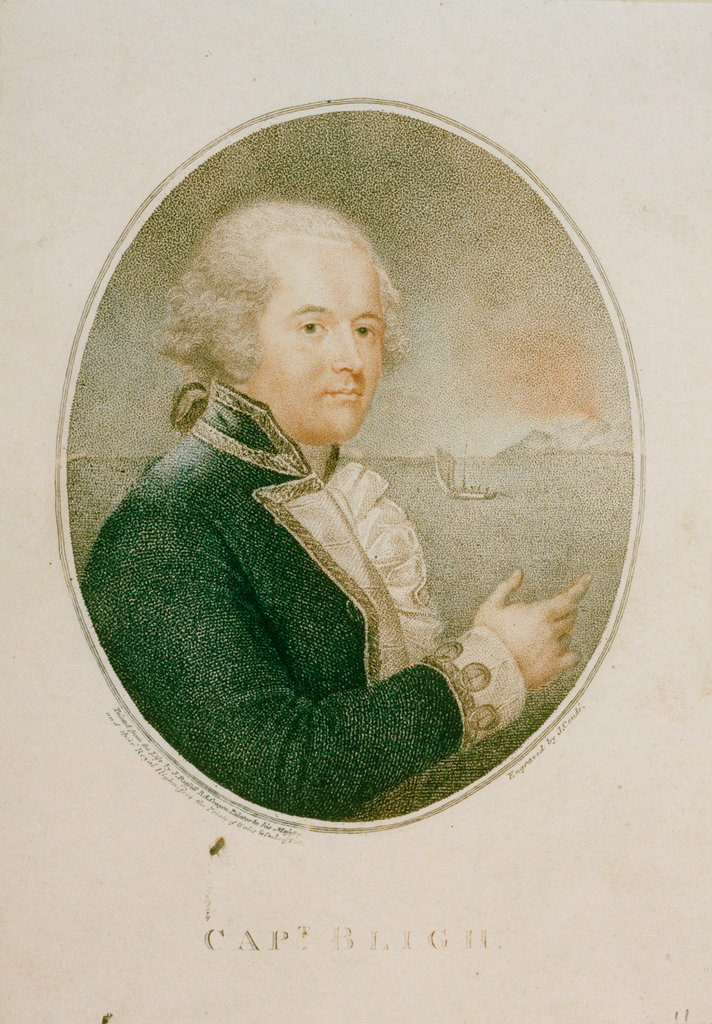The image is a detailed engraving of the notorious Captain Bligh from Colonial times. It is housed within an oval frame centered on a light brown, slightly pinkish rectangular background. The entire piece measures approximately six inches tall and three inches wide, with the oval itself being about three inches high and two and a half inches wide, bordered by a very light brown edge. 

The central figure, Captain Bligh, depicted from the mid-waist up, commands attention with a prominent, full face, marked by a straight nose and a slight double chin. His white hair, brushed back and curled at the sides in the fashion of his time, is tied into a small ponytail at the back. He is adorned in an old-fashioned captain's uniform, a dramatic ensemble of a bluish-brown or bluish-black high-collared seacoat, featuring a white ruffled shirt underneath and ornate cuffs accentuating his sleeves. His right arm is bent, with his hand extended forward, gesturing toward the sea, perhaps in the throes of recounting a tale of mutiny.

In the background, behind Captain Bligh, lies a vivid maritime scene: an open bay with a single-masted sailboat calmly set against an island ghosted in the distance. To the right, a mountain ominously spews red and black smoke, adding an element of dramatic tension to the serene sea. Beneath the oval frame, there is some small, curved, unreadable writing, while prominently, in larger letters, it is inscribed, "CAPT. B-L-I-G-H." The engraving is credited to J. Calm, identified by text to the lower left of the oval. 

Overall, the image exudes a tan hue, resonating with antiquity and echoing the illustrious and tumultuous maritime legacy of Captain Bligh.